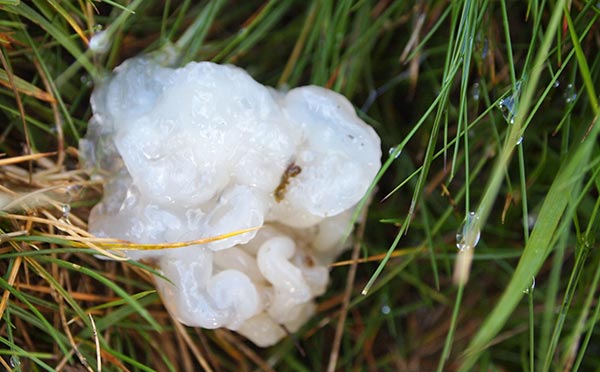This photograph captures a close-up of a grassy area dominated by a peculiar, white, gelatinous glob. Positioned prominently in the frame, this semi-transparent, blobby substance is surrounded by thin, green blades of grass with delicate water droplets clinging to them, especially on the right side of the image. The glob's texture is complex and uneven, resembling either a cluster of insect eggs or chewed-up gum. It has a shiny, wet surface that reflects light, contributing to its worm-like appearance. To the left, the grass appears more dried and yellowed, contrasting with the lush green surrounding it. A notable feature within the glob is a small piece of brown dirt embedded in its upper right section, adding to its mysterious nature. The photo overall highlights the intriguing contrast between the wet, reflective blob and the diverse textures of the dewy grass and dried blades around it.